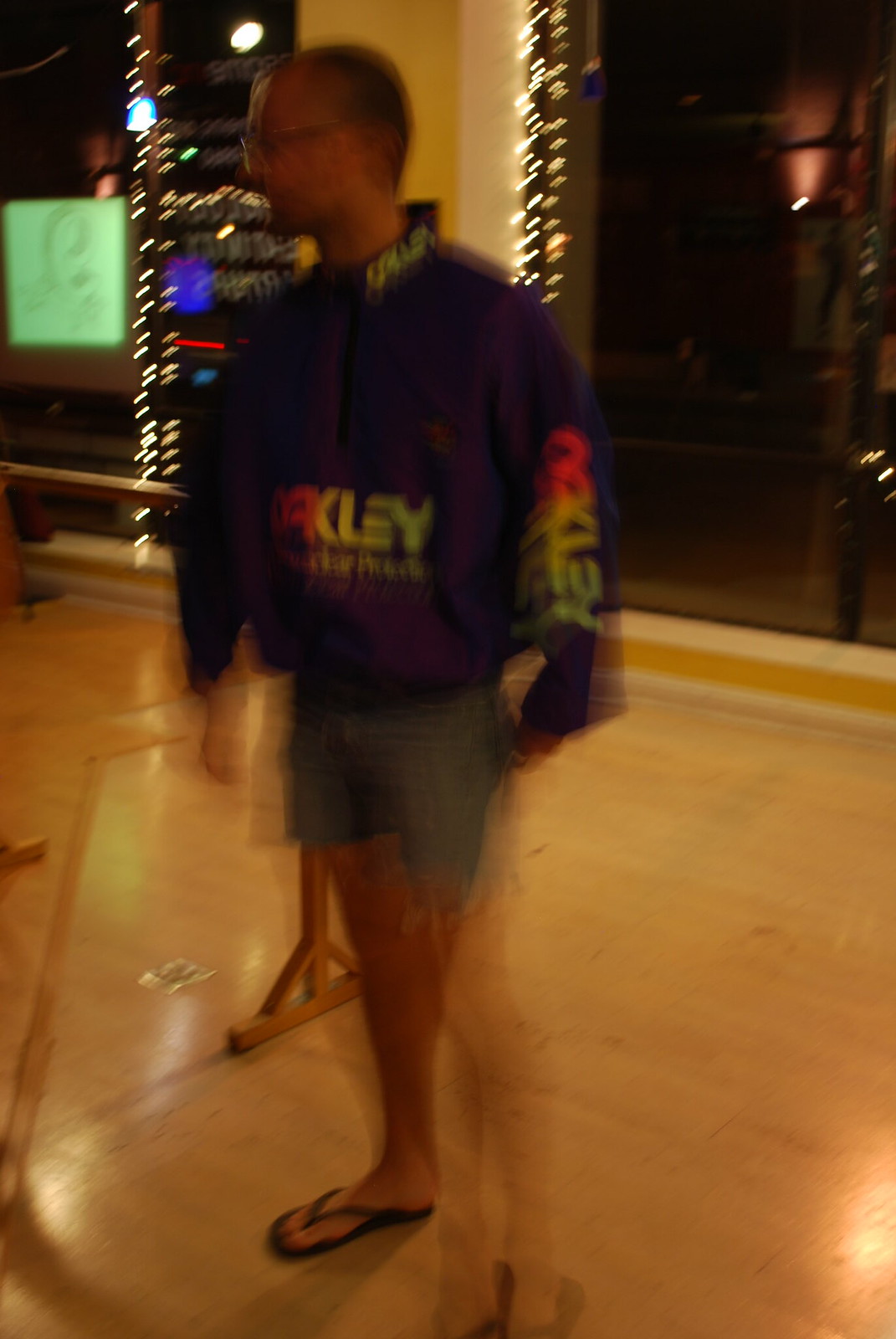In this blurry, dimly lit vertical frame, the image portrays a cozy interior scene bathed in a yellowish hue. The image is poorly lit, giving it a somewhat nostalgic and subdued atmosphere. A light tan wood grain floor adds warmth to the setting. A man, who is the focal point of the image, stands at a slight angle facing towards the left side of the frame. He is dressed in a long sleeve black shirt emblazoned with the word "Oakley" across the chest, with the letters blending from red to yellow to green. Complementing his casual attire, he wears dark green shorts and black flip flops, adding to the laid-back ambiance of the scene.